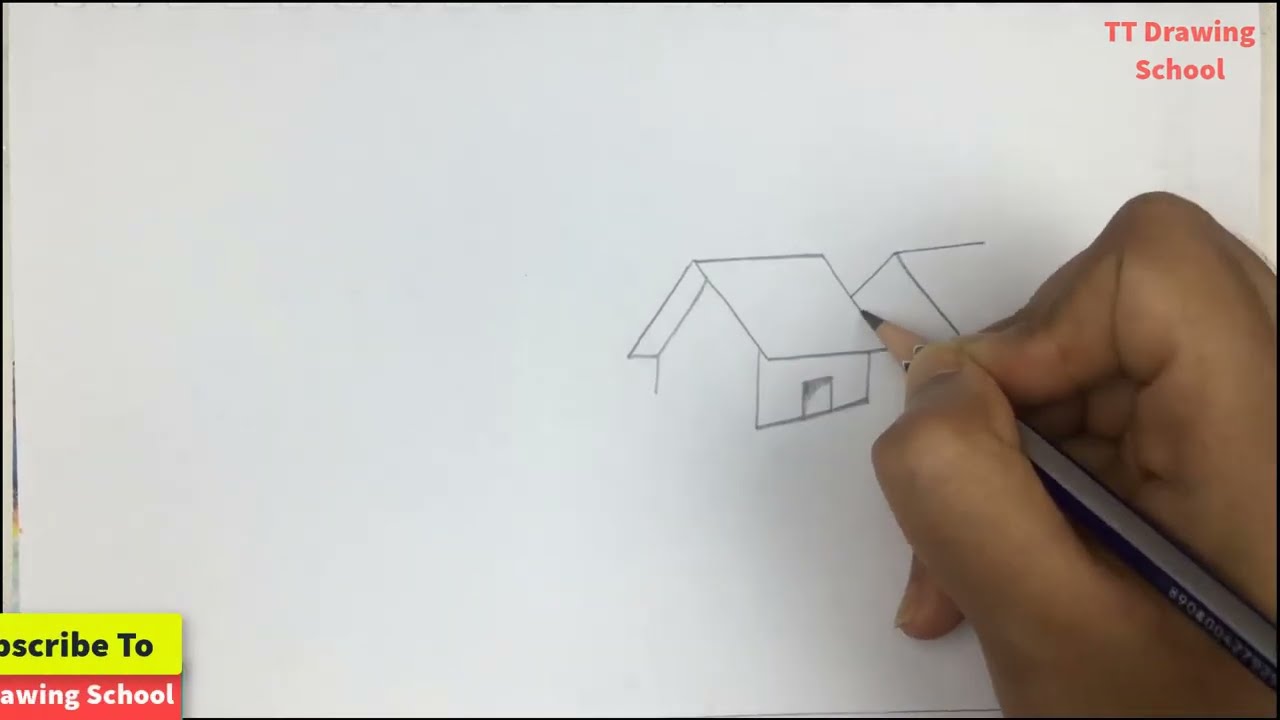In an image titled "TT Drawing School" displayed in red at the upper right corner, a dark-skinned human hand, positioned at the bottom right, holds a sharp black pencil and draws on a white sheet of paper. The artist has completed one house with a triangular roof and a single door positioned centrally in the image. They are currently sketching the rooftop of a second house to the right of the first. The scene captures the meticulous rendering of what appear to be 3D-like houses. Additionally, at the bottom left, there is a prompt that says "Subscribe to" in black text on a yellow rectangle, followed by "Drawing School" in white text on a red rectangle.